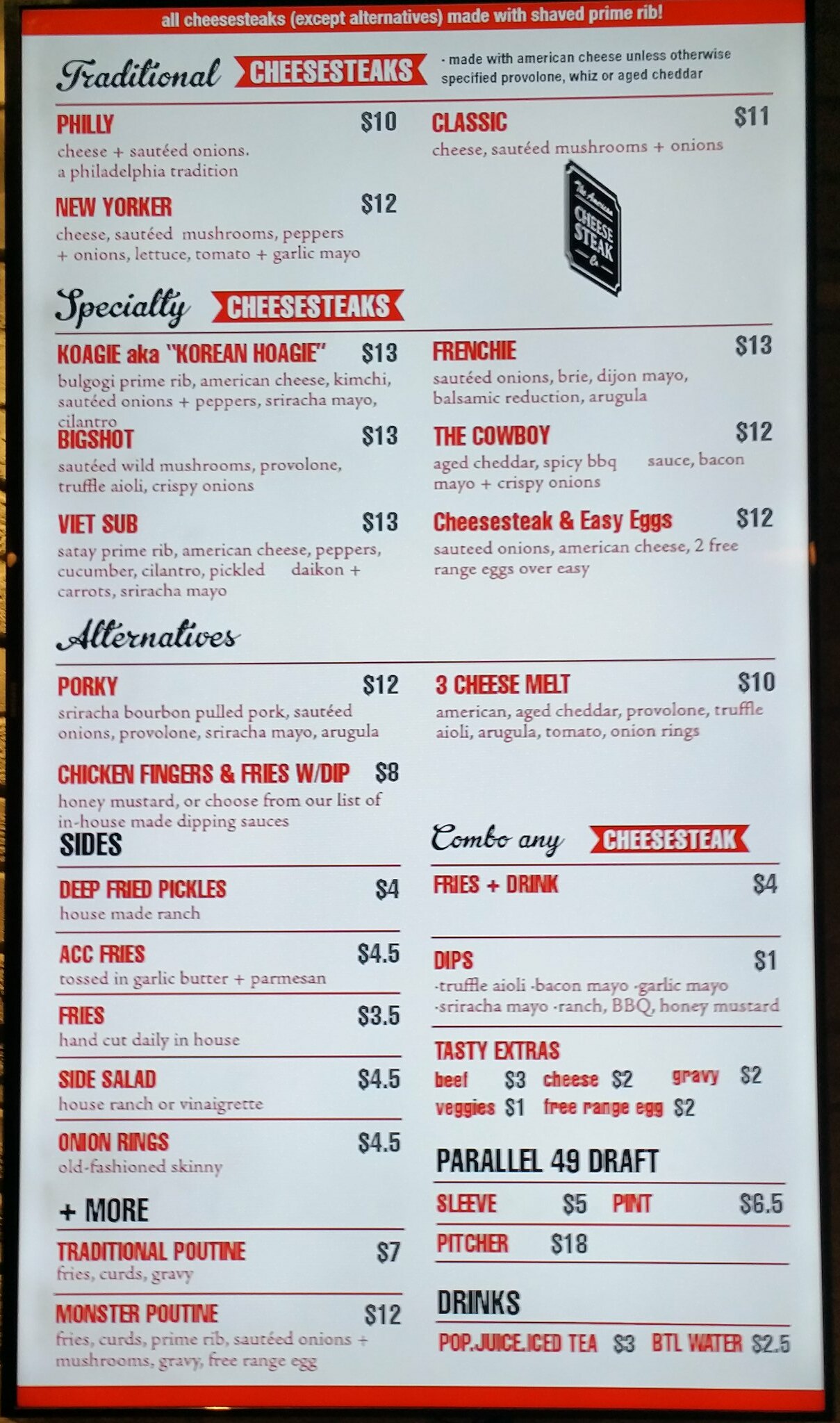A meticulously organized menu at a restaurant is displayed in a long rectangular shape, significantly longer than it is wide. At the very top, a red border frames the header, which reads "Cheese Steaks" in white lettering, with a subtitle noting that alternatives are made with shaved prime rib.

The menu is divided into two columns: left and right.

### Left Column:
1. **Traditional Cheesesteaks** (in red)
   - Listings Include:
     - Philly
     - New Yorker
   - Each item’s name is listed on the left with the price in red on the right.

2. **Specialty Cheesesteaks** (title in black)
   - Listings Include:
     - Three specialty cheesesteaks, each priced with the amounts in red on the right.

3. **Alternatives** (title in black)
   - Listings Include:
     - Deep-fried pickles (listed items with prices in red to the right)
   - There are two options under this section, each priced at $12.

4. **Sides** (title in black)
   - Listings Include:
     - Five different sides, each named and priced in red to the right.

5. **Plus More** (last section on the left side in black)
   - Listings Include:
     - Two additional items, names in red with prices to the right.

### Right Column:
1. **Combos** 
   - Listings Include:
     - Cheesesteak Combo
     - Other combo options (each with details and prices in red to the right).

2. **Tasty Extras** (title in black)
   - Listings Include:
     - Five additional items, each listed with the price in red to the right.

3. **Parallel 49 Draft** (subsection in black)
   - Listings Include:
     - Three draft options, each detailed with specific names and prices in red to the right.

4. **Drinks** (at the bottom)
   - Listings Include:
     - Pop
     - Juice
     - Iced Tea
     - Bottled Water

The menu is bordered at the bottom by a red line, creating a pleasing symmetry with the top border. The entire menu's center remains white, making the text and various sections clear and easy to read.